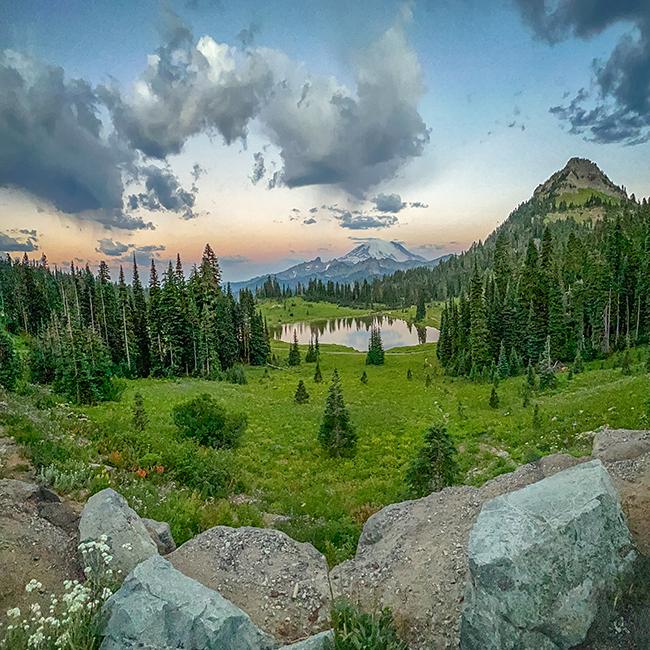The image depicts a stunning outdoor scene that seems to be in a park or a natural reserve, featuring a tranquil lake that resembles a sheet of glass. The vantage point is from a spot behind a rock formation or rock wall in the foreground, leading down a small hill with a weedy field scattered with trees. A trail meanders through this section and around the lake, framing the serene water bordered by an array of lush, evergreen trees.

To the right side of the lake and extending around to the left, there's a continuous tree line marking the beginning of a dense forest. The landscape transitions into grassy meadows on both sides of the lake, eventually leading up to a taller, imposing mountain in the distance. Behind these features, the sky displays hues of blue, orange, and pink, indicating either sunset or sunrise, adding an enchanting glow to the scene. The high-peaked mountains in the background and a closer mountain to the right further enhance the depth and majesty of the environment. Overall, it's a picturesque, verdant valley area with a tranquil, reflective lake at its center, nested within a lush, vibrant, and expansive natural landscape.